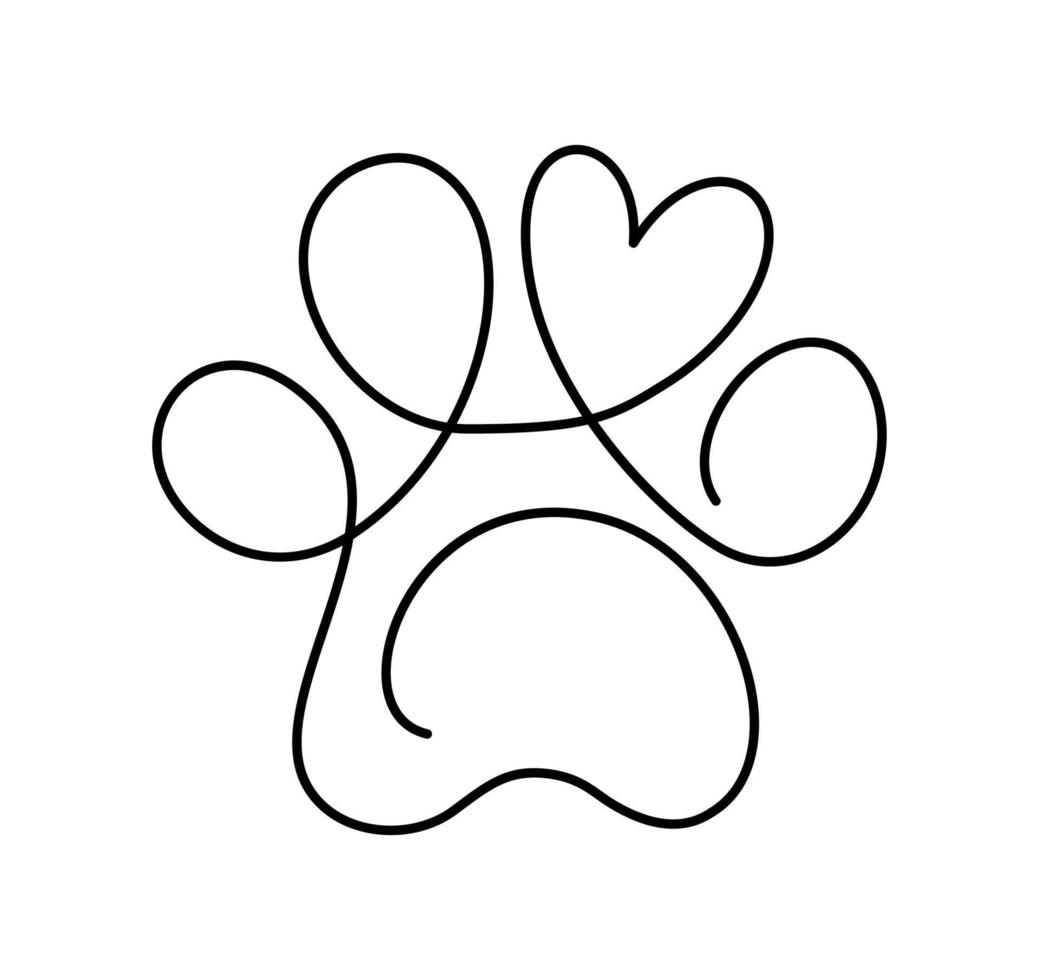This image features a digitally created, intricate line drawing made from a single, thick black line against a white background. The continuous line curves and loops back on itself, forming a shape reminiscent of an animal's paw, such as that of a cat or a dog, though it is not an exact representation. Notably, near the top right of the drawing, one of the loops forms a heart shape. The drawing is not symmetrical, but it exhibits a certain pattern and predictability, with two curved portions on the left and right in the middle. Despite its simplicity, the design showcases a blend of artistry and digital precision.